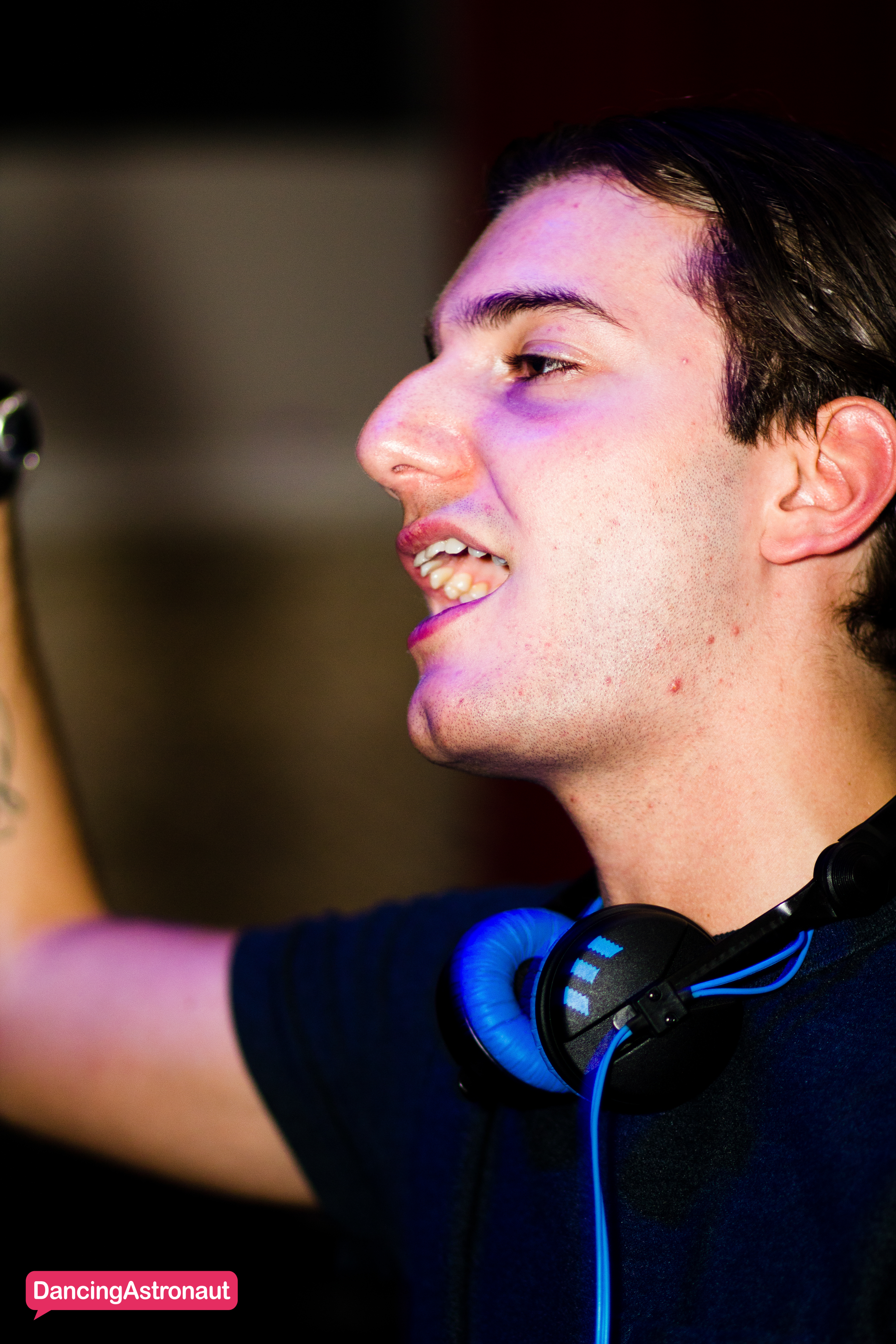The image is a close-up view of a man seen from the chest up, positioned towards the right side of the frame and facing to the left. He has short dark hair, very short stubble, and a cleft chin, giving him a distinctive profile. His mouth is open, revealing his teeth and part of the roof of his mouth, and he has a unique nose. He is raising his right arm, which stretches all the way to the left side of the image, adorned with a wristwatch. A tattoo is partially visible on his forearm. 

He is wearing a dark blue, short-sleeved t-shirt and has a pair of black and blue over-the-ear headphones around his neck. The headphone wires are light blue, matching the interior cushion. The background behind him is completely out of focus, rendered in a dark, brownish tone. At the very bottom left corner of the image, there is a small thought bubble in red and white with the words "Dancing Astronaut."